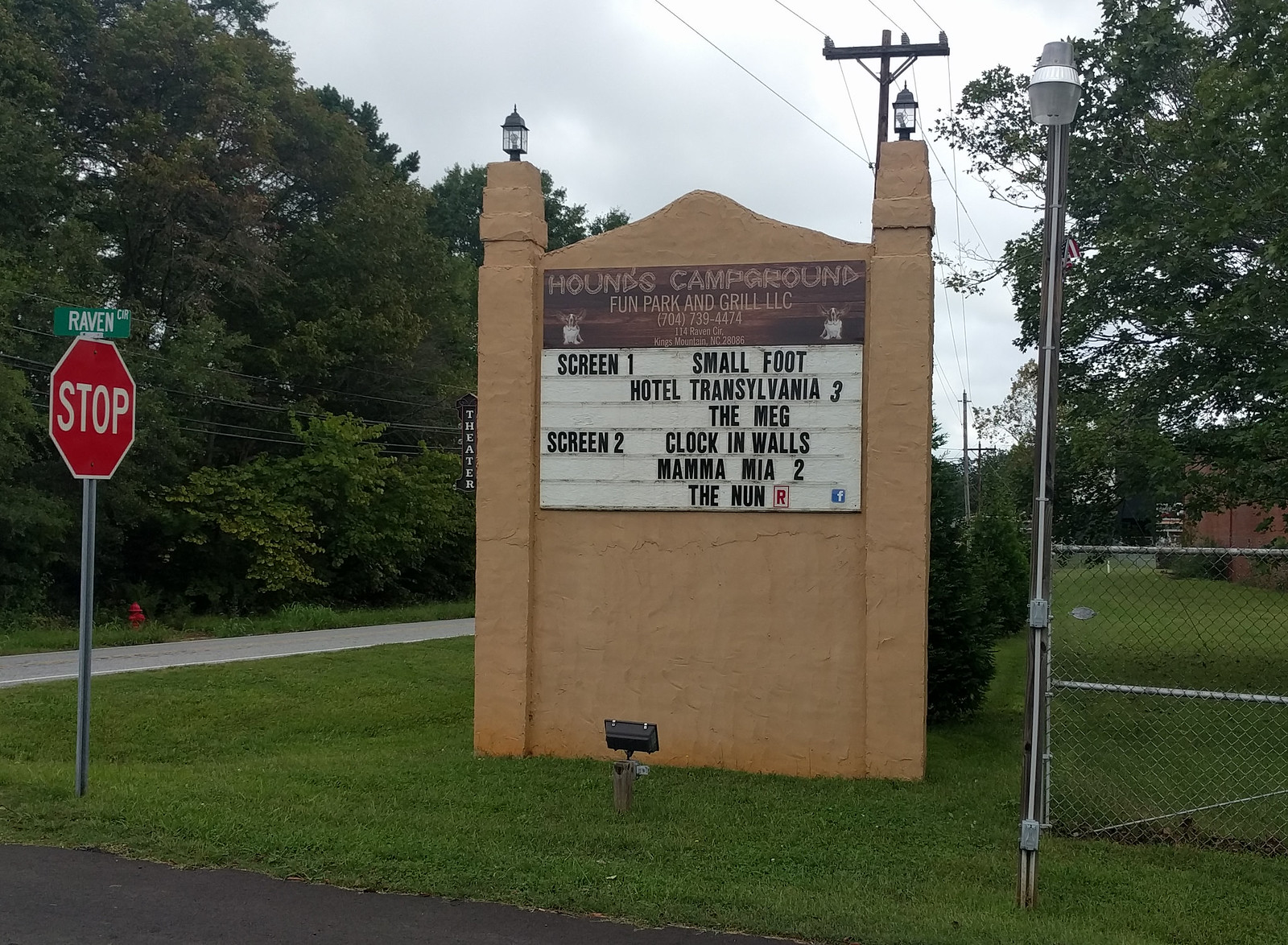This outdoor photograph captures a street corner where a stop sign and a green roadway sign displaying the word "Raven" in white letters are prominently visible. Adjacent to these is a tall, stone sign structure, enclosed by a metal fence, indicating the presence of the Helms Campground Fun Park and Grill LLC. The top section of this sign is dark with white 10-letter text stating "Helms Campground." Below this, a theater marquee in white letters lists current movies: on Screen 1, "Smallfoot," "Hotel Transylvania 2," and "The Meg," while Screen 2 shows "The Clock in the Walls," "Mamma Mia 2," and "The Nun," which includes a red Rated-R symbol. Additionally, there's a small black light fixture intended to illuminate the sign at night, though the photo is taken during the day.